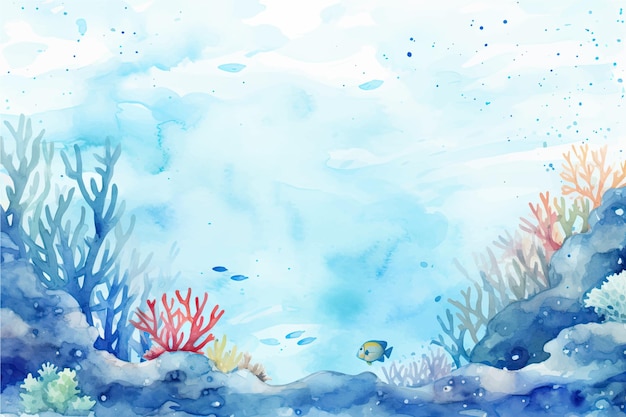This watercolor painting beautifully captures an undersea scene in a horizontal rectangular frame. The predominant palette is a mesmerizing blend of blues, teals, and aquas with splashes of red and gold. At the bottom of the frame, the ocean floor is depicted in various shades of dark blue, adorned with an array of coral formations—primarily bluish but including vibrant pieces of red and a striking goldish coral. Rocks interspersed with algae and plankton, in hues of blue, red, gray, orange, and green, add texture and depth to the composition.

In the foreground, a vividly colored yellow fish with blue trim swims to the left, becoming the focal point against a backdrop of a gradient blue sea. Smaller blue fish silhouettes can be seen scattered throughout the mid and distant background, enhancing the sense of depth and movement. The water above is a symphony of swirling blues, accented by white patches that resemble clouds, creating a serene and immersive underwater atmosphere. The overall effect is a harmonious and detailed portrayal of the ocean's rich and diverse ecosystem.